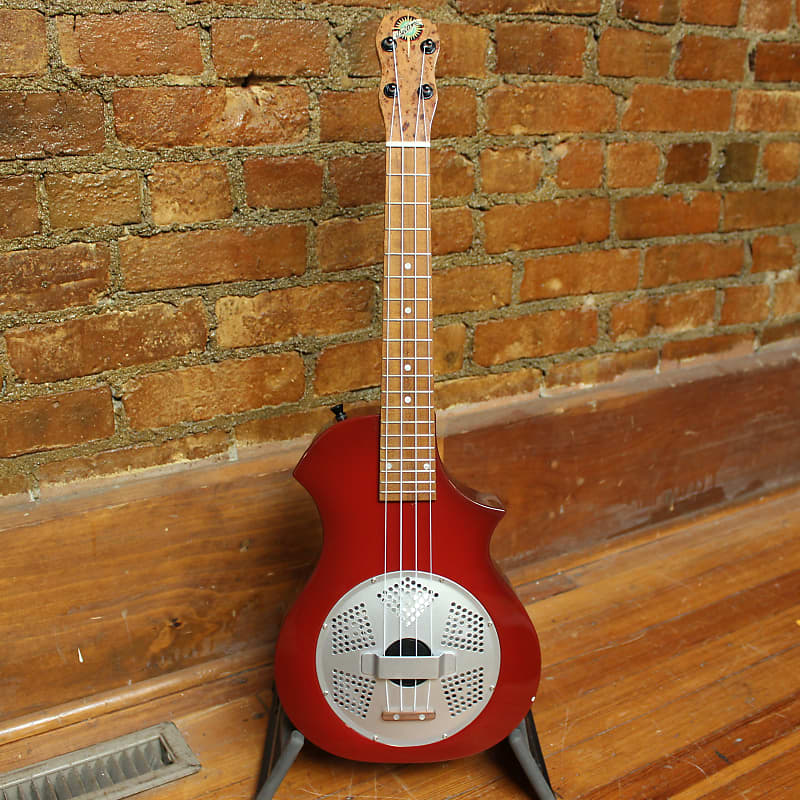This color photograph captures a striking red bass guitar standing upright on a black and gray stand, placed on a wooden floor. The scene is set against a backdrop of a red brick wall, which is partially covered by a wooden baseboard running the length of the wall. In the lower left-hand side of the image, a metal vent is visible. 

The red guitar features a prominent large silver circle in the center, surrounded by vent-like holes. The guitar has four well-defined strings stretching up its brown wooden neck, which is adorned with silver frets and terminated by black knobs. At the top of the neck, there is an intriguing, star-shaped logo in black, gold, and green, although the specific details are not fully readable. The overall unique design, including the circle with holes, contributes to the guitar's distinct appearance.